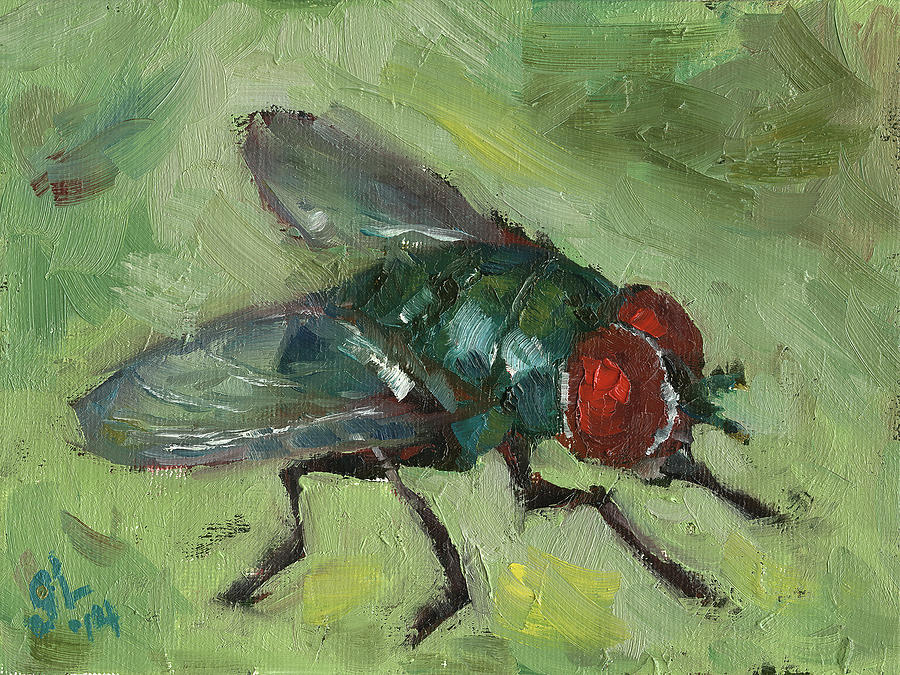This oil painting features a fly prominently centered within a horizontal rectangle canvas that's about 1.5 times as wide as it is tall. The fly, facing to the right, boasts big red eyes, six dark legs, and a dark green body. Its wings are depicted as translucent with a blend of blue, green, and silver hues that allow the viewer to see parts of its body underneath. The background is primarily composed of broad, wavy brush strokes in various shades of green, ranging from light to dark, with touches of yellow and a small hint of red in the upper left corner. In the bottom left, the artist's signature, “gL 14,” is painted in blue, indicating the initials GL and the year 2014. The brushwork throughout is crude yet expressive, giving the painting an abstract, dynamic feel.